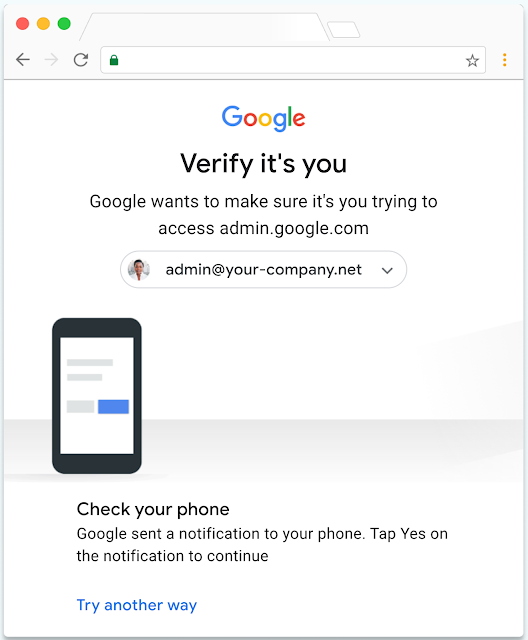A screenshot of a Google verification window is depicted. The window is from the Google security checkup, ensuring the user is genuinely trying to access an admin account, either at admin.google.com or at admin.yourcompany.net. The interface features several elements: red, yellow, and green status indicators, left and right arrows, a refresh button, and a green lock icon. A holographic star symbol is also present. Google prompts with the message: "Verify it's you. Google wants to make sure it's you trying to access admin.google.com or admin.yourcompany.net." Below this message, a dropdown menu appears, indicating that a notification was sent to a smartphone with black edges. Users are instructed to check their phone and tap "Yes" on the notification to continue. Alternatively, they can choose to "Try another way." The window also includes gray bottom lines and blue edges, consistent with the theme of the browser interface.